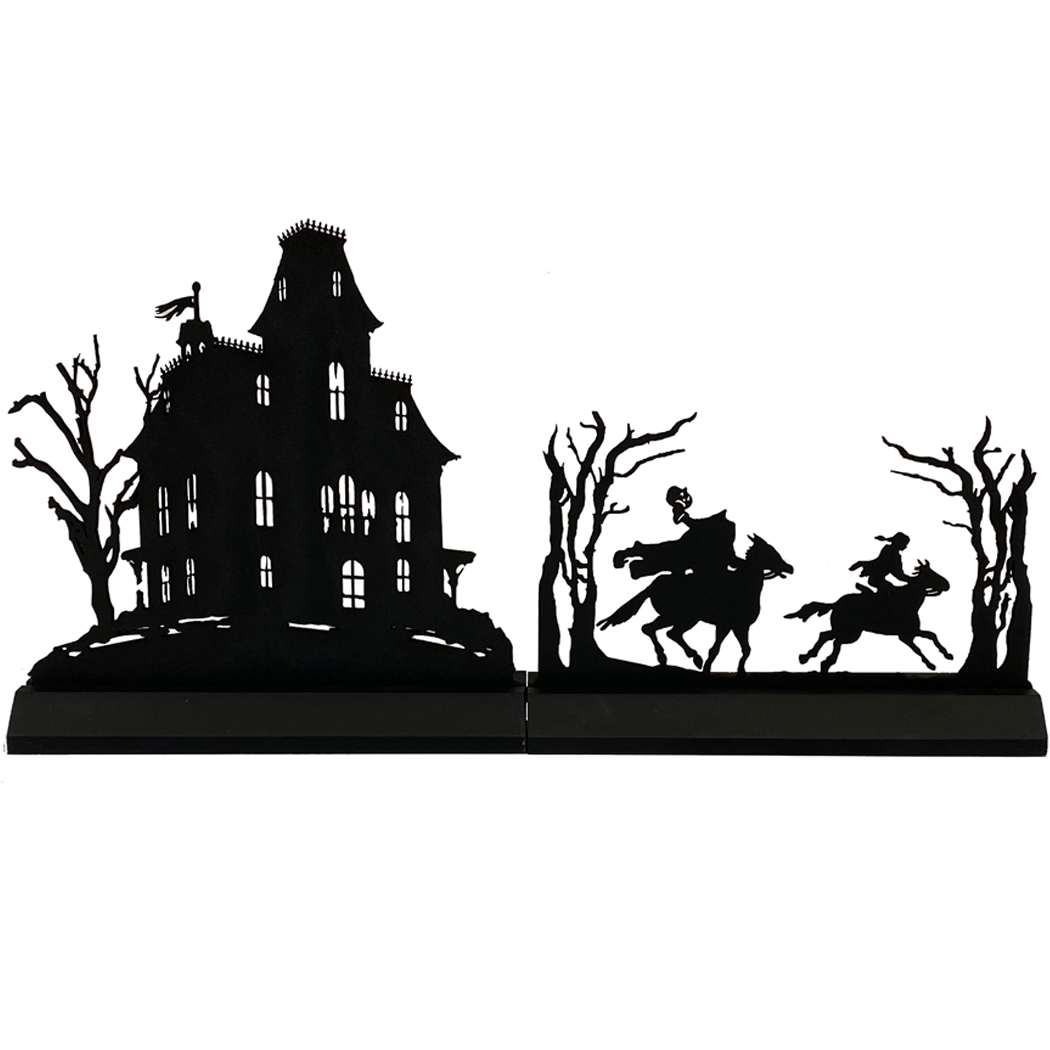The black and white image depicts a 3D silhouette scene spread across two platforms with detailed cutouts. On the left platform, there is a large Victorian-style manor with arched windows, a steeple with a flag, and a dead tree bereft of leaves, standing against a pure white background. The right platform features a chilling chase scene: the Headless Horseman galloping, holding a carved pumpkin jack-o'-lantern high in his right arm, pursuing a panicked Ichabod Crane on a smaller horse. This macabre scene, set within a wooded area of barren, leafless trees, captures the eerie essence of Sleepy Hollow.